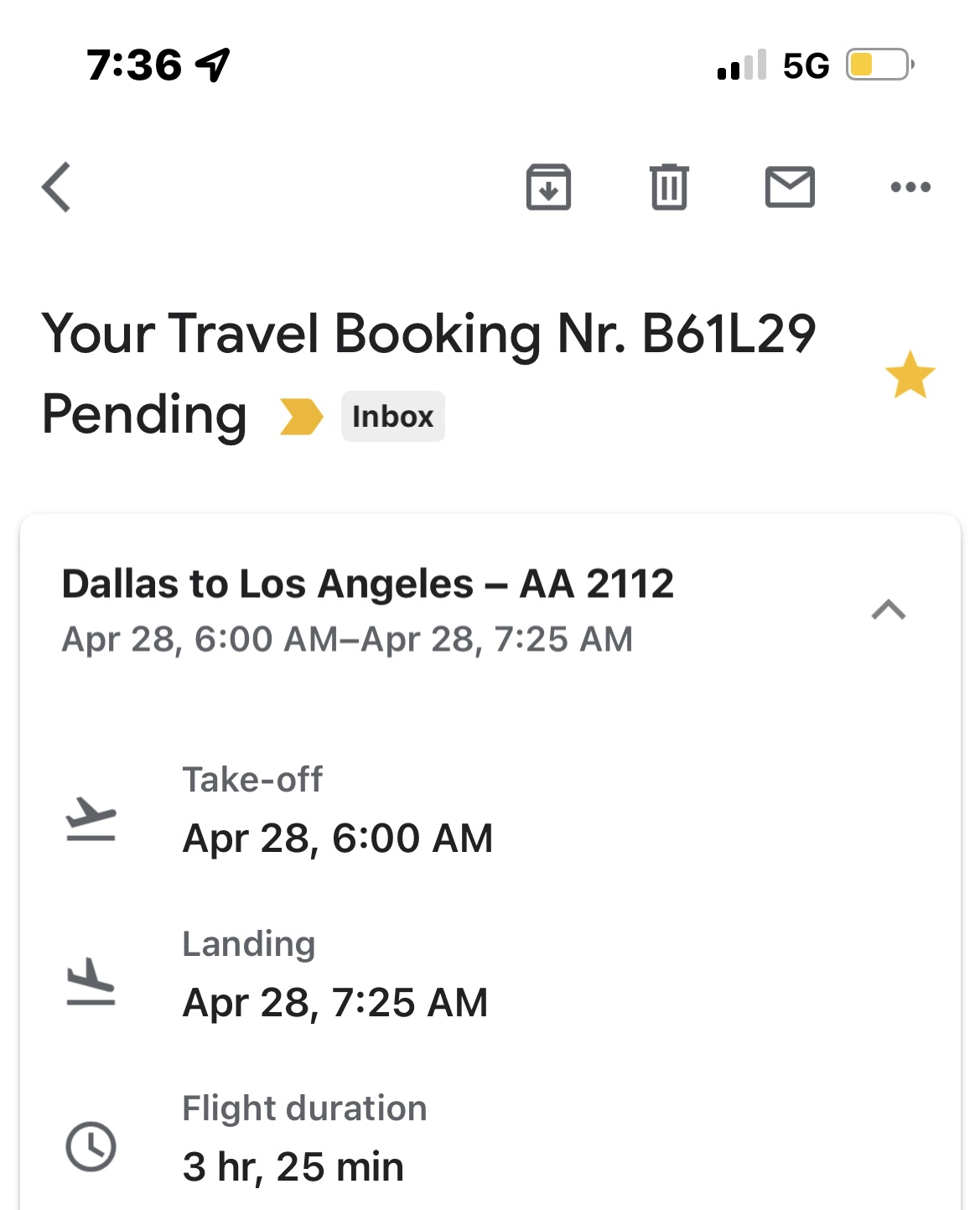A screenshot of an email on an iPhone is depicted. The interface shows various elements common to an email composition or viewing screen. At the top left, "7:36" is displayed in black Arial font, indicating the current time. Towards the right of the time stamp, a right-pointing navigation icon is outlined in black, followed by the mobile signal strength showing 2 out of 4 bars. Next to it, "5G" indicates the network connection, and further to the right, a battery icon in yellow signifies that the device is in low power mode with approximately one-third battery remaining.

Directly below this status bar, a gray arrowhead pointing to the left is visible, indicating the option to return to the previous menu. Adjacent to this arrowhead, a 3D-effect button is depicted with a downward-pointing arrow on it, possibly for minimizing options. Towards the right side of this are three icons: a trash can for deleting the email, an envelope symbol, and three vertical dots suggesting additional settings or menu options.

The subject line of the email reads "Your travel booking rB61L29 pending" in black text. Below the subject, a yellow tag symbol is displayed alongside a light gray rectangle containing the word "Inbox" in bold black writing. On the far right side of this gray rectangle is a filled orange star icon.

In the body of the email, a rounded, shadowy, gray-bordered rectangle indicates booking details. The top left of this section shows "Dallas to Los Angeles - AA2112" in bold black lettering. To the right, a gray arrowhead points upwards. Below this, the departure and arrival times are stated in gray: "APR 28, 6:00 AM - APR 28, 7:25 AM".